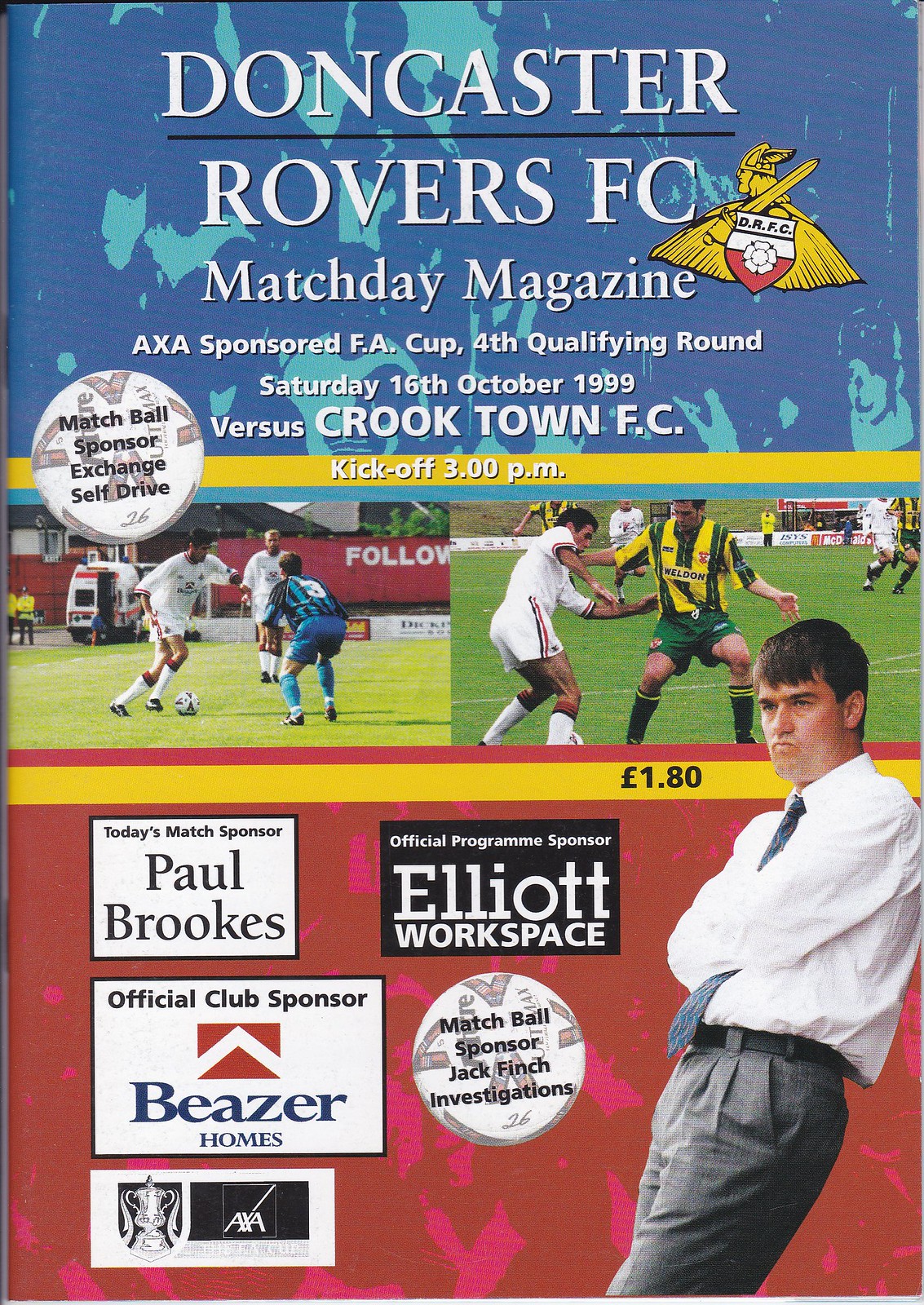The front cover of the Doncaster Rovers FC matchday magazine for the FA Cup fourth qualifying round, sponsored by AXA and dated Saturday, 16th October 1999, prominently features dynamic images from two different soccer matches. In the lower right corner, a stern-looking coach stands with his arms crossed, dressed in a long-sleeve white shirt and gray pants. Beside him, the official sponsors' logos are neatly arranged in square boxes, showcasing Paul Brooks, Beezer Homes, Elliott Workspace, and Jack Finch Investigation.